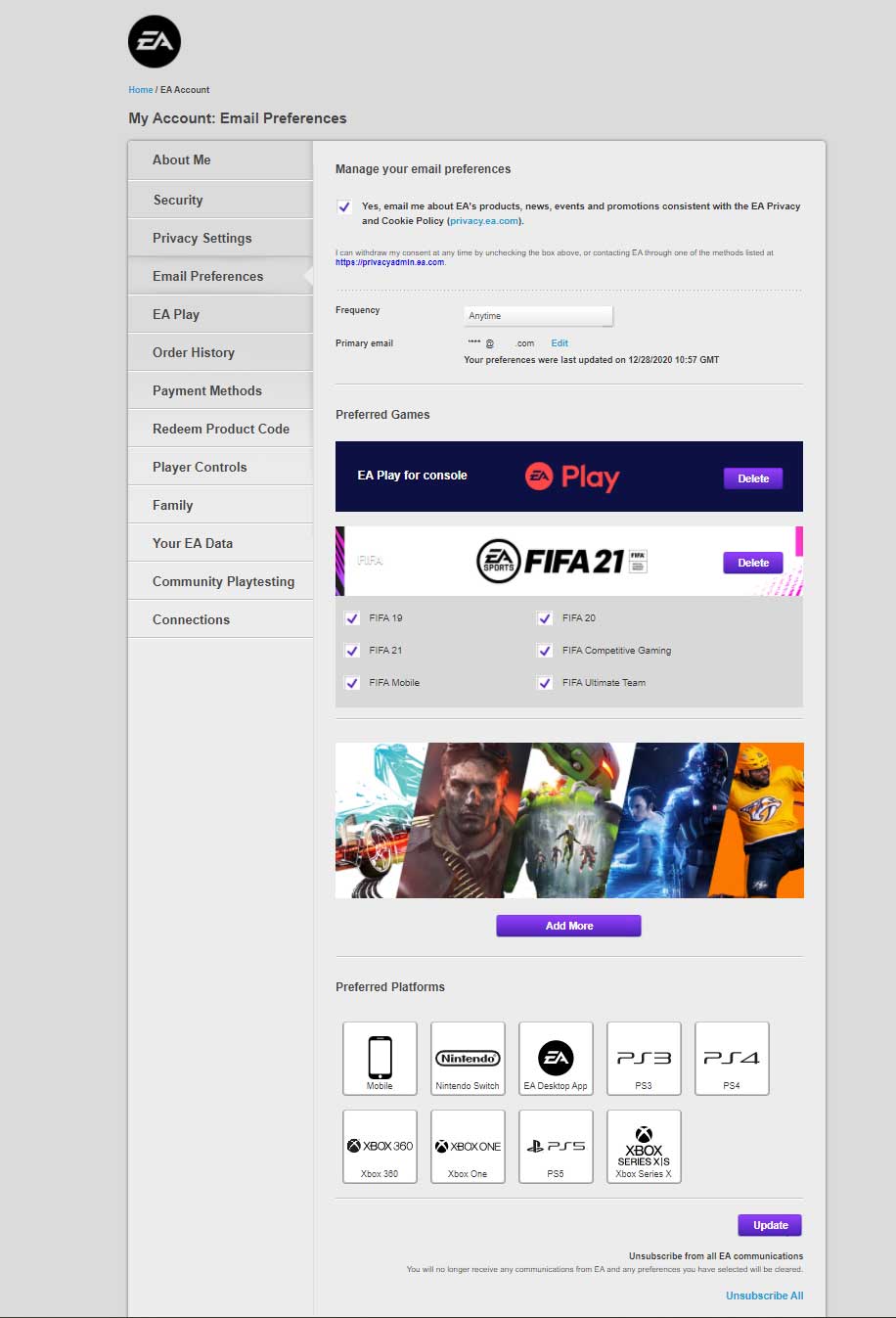In this detailed screenshot from an EA Sports video game interface, the user is navigating through EA Account settings at the top, where options such as "Home" and "Blue" are visible. The focus is on the "Email Preferences" section visible on the left-hand side menu, which includes other options like "About Me", "Security", "Privacy Settings", and more.

Within the Email Preferences section, users can manage their email subscriptions by selecting checkboxes for EA Products, Events, News, and more. There is a cookie policy segment and an option to choose the frequency of emails received. Below this, the primary email address is displayed, with the last edit date of 12-28-2020, and an option to edit it if necessary.

The user can also specify preferred games such as "EA Play for Console" and manage or delete these preferences. Games like "FIFA 21" have a dedicated section where users can check boxes for different versions such as FIFA 19, 20, 21, as well as categories like competitive gaming, mobile, and ultimate team.

A series of images feature various EA Sports games, including a racing game, potentially "Call of Duty", and an NHL game. There is a button to add more games to the list. Platform-specific images for Xbox One, PS5, and EA Sports are also present. An "Update" button is prominently displayed at the bottom, along with an option to "Unsubscribe All" in blue.

The left-side menu also includes comprehensive sections like "Order History", "Payment Method", "Redeem Product Code", "Player Controls", "Family", "Your EA Data", "Community Playtesting", and "Connections".

This caption intricately describes the elements visible in the user interface, giving a clear view of how to navigate and manage the EA Account settings specifically related to email preferences.